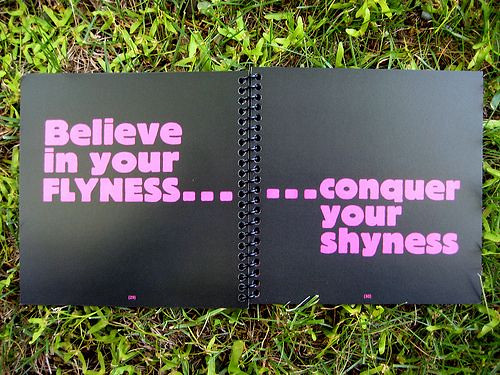The image showcases a vibrant scene of lush, wild-growing, green grass with an open black spiral-bound notebook placed on it. The notebook's cover features bold, pink writing in a heavy, thick font. On the upper left-hand corner of the cover, the phrase "believe in your flyness..." is printed, with the ellipses rendered as small rectangles. On the lower right-hand corner, completing the motivational quote, it reads, "conquer your shyness." The black wiring of the spiral binding is clearly visible, segmenting the notebook. There is also some tiny, unreadable pink text at the bottom of each page. The contrast of the vivid green grass and the black notebook with striking pink text creates an eye-catching and inspirational scene.